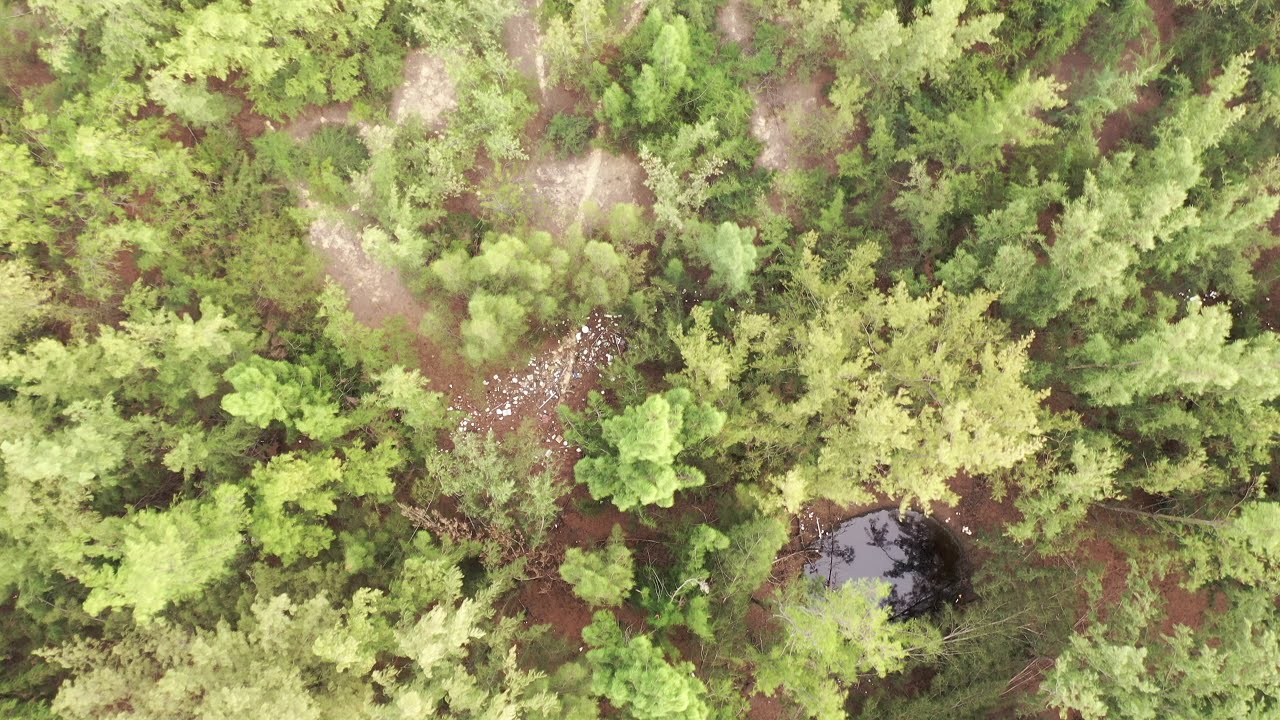The image is an aerial photograph captured from a top-down perspective, showcasing a densely wooded area that is abundant with a variety of trees, some with light green foliage and others that appear to be pine trees. The ground below is covered in various shades of brown and red, likely composed of dirt, fallen leaves, and pine needles, giving it a rough, rocky, and earthy appearance. Scattered throughout the forest, there are numerous dirt trails winding through the trees, notably visible in the upper left-hand side of the image. In the lower right-hand corner, there is a small, perfectly round pond with a deep greenish hue, its still waters reflecting the surrounding treetops. The scene is captured in broad daylight, providing a clear and detailed view of this tranquil natural landscape.